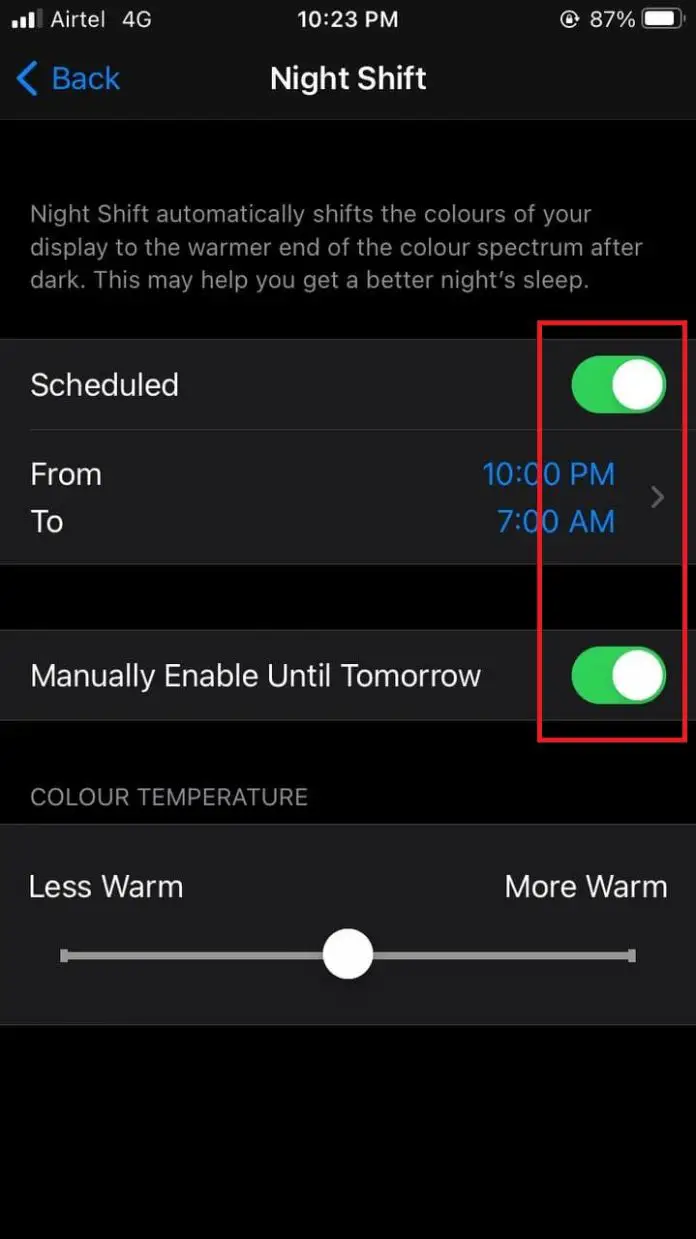This is a detailed screenshot of a mobile phone screen featuring a Night Shift settings interface. The background is black with white text. 

In the top left corner, icons display signal strength and "Airtel 4G." Centrally positioned at the top is the time, "10:23 PM." On the right side, there is a clock icon followed by the battery status, showing "87%" next to a white battery icon.

Beneath this status bar, the interface begins with a blue back arrow and the word "Back" on the left side, and "Night Shift" at the center. Below the title, there is descriptive text: "Night Shift automatically shifts the colors of your display to the warmer end of the color spectrum after dark. This may help you get a better night's sleep."

Following this description, the label "Scheduled" appears. To the right, a green slider indicates that the scheduling feature is enabled. Beneath, the schedule "From 10 PM to 7 AM" is listed, with "10 PM" in blue. Further down, the option "Manually Enable Until Tomorrow" is also shown with a green slider turned on.

A red rectangle outlines the section that includes these two sliders and the specified times, possibly to highlight this area for discussion.

At the bottom, the setting "Color Temperature" is listed alongside a white slider. The slider ranges from "Less Warm" on the left to "More Warm" on the right, with the indicator dot set directly in the center.